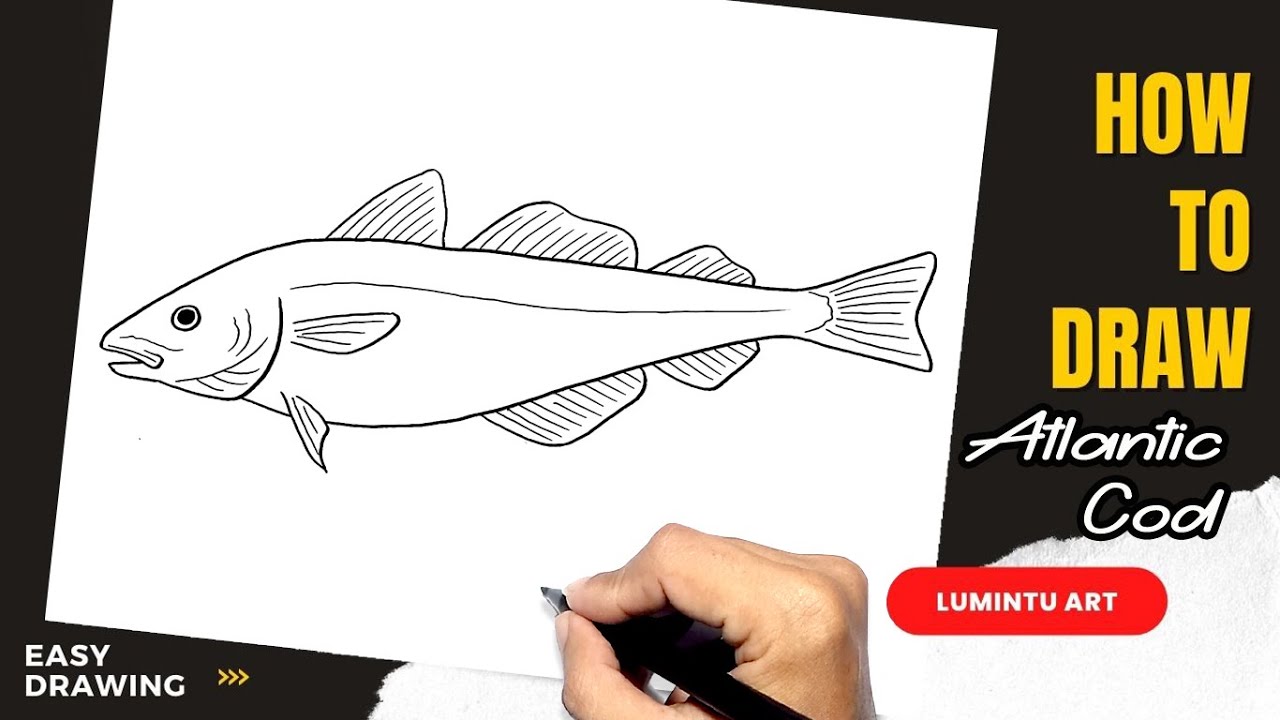The image features a color photograph of a hand holding a black ink pen, drawing a line art illustration of a fish on what appears to be thick white paper. The fish, depicted in black and white as line art, somewhat resembles a trout but lacks any color details, making it difficult to identify the species definitively. The setting is against a black background. Text elements include "Easy Drawing" in white, situated in the lower left corner against the black background with three small yellow arrows pointing right. In the upper right, large yellow text reads "How to Draw," and below that, in white text with a black outline, it says "Atlantic Cod." Additionally, a red oval in the lower right corner, partially overlapping the main white drawing paper, contains the white text "Lumenti Art." The overall layout of the poster is in landscape orientation.